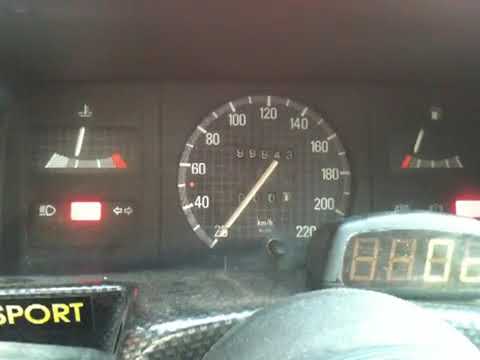The image shows a detailed view of a car's dashboard, predominantly featuring the speedometer that reads at zero. To the left of the speedometer, various indicator lights can be seen, including a lit check engine light, a headlight indicator, a turn signal light, and an engine heat indicator. Notably, the check engine light is illuminated. On the right side of the speedometer, there's a fuel gauge indicating the tank is nearly empty, along with additional engine lights, including a brightly lit engine light. Below the speedometer, a digital speedometer also reads zero. On the bottom left corner of the display, the word "SPORT" is clearly visible in yellow. To the right, partially visible, is the top section of the steering wheel. Additionally, the speedometer itself features an analog dial ranging from 20 to 220 mph, and there is an odometer showing approximately 99,000 miles. The trip meter has been reset, and the temperature gauge is a quarter into the hot zone. The lower right section of the dashboard displays a reading of "8888," potentially indicating RPMs or another metric, further suggesting that this dashboard belongs to a sport or race car.